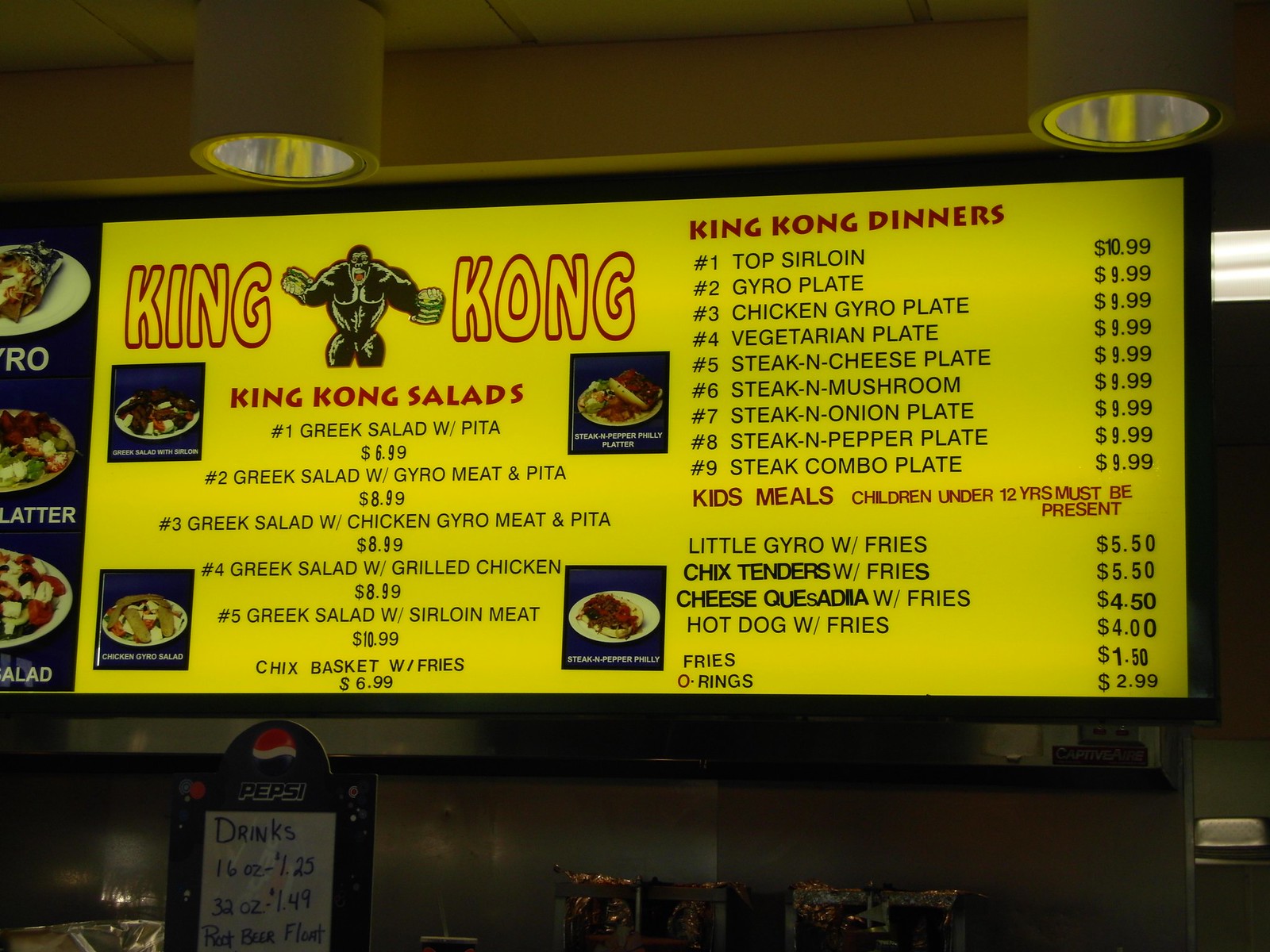This is a vibrant color photograph showcasing a menu from King Kong, a restaurant with various meal options. The menu is prominently organized under several headings: "King Kong Salads," "King Kong Dinners," and "Kids Meals." 

Under "King Kong Salads," the offerings include:
- Greek Salad with Pita
- Greek Salad with Gyro Meat and Pita
- Greek Salad with Chicken Gyro Meat and Pita
- Greek Salad with Grilled Chicken
- Greek Salad with Sirloin Meat
- Chick's Basket with Fries

The "King Kong Dinners" section features:
- Top Sirloin
- Gyro Plate
- Chicken Gyro Plate
- Vegetarian Plate
- Steak and Cheese Plate
- Steak and Mushroom Plate
- Steak and Onion Plate
- Steak and Pepper Plate
- Steak Combo Plate

For the younger diners, the "Kids Meals" section stipulates that children under 12 years must be present to order. The options include:
- Little Gyro with Fries
- Chick's Tenders with Fries
- Cheese Quesadilla with Fries
- Hot Dog with Fries

At the bottom of the menu, there is an additional section for "Fries and Onion Rings."

The menu is adorned with appetizing photos of some of these dishes. The entire sign is set against a bright yellow background, capturing attention with an image of King Kong prominently displayed at the top, adding a playful and themed touch to the overall design.